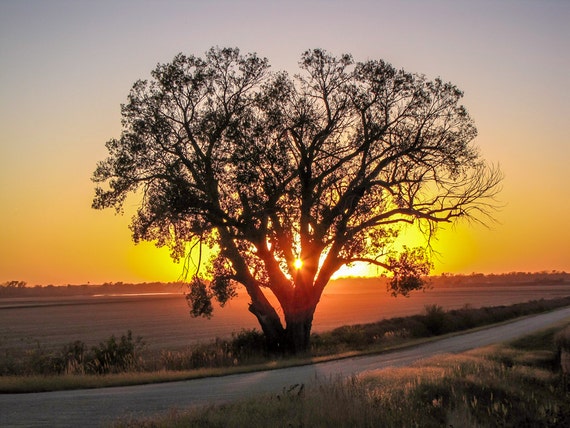The photograph captures a serene countryside scene with the focus on a massive tree standing by an asphalt gravel road. The rising sun, positioned behind the tree, casts gorgeous golden hues and vibrant shades of orange, pink, and yellow across the sky, illuminating the scene with a peaceful, ethereal light. The sun's rays filter through the tree's branches, creating a striking silhouette. There are no people or animals around, contributing to the tranquil atmosphere. The backdrop of the image reveals a farm field that appears to have been recently cropped, enhancing the rustic charm of the scene. The overall composition evokes a sense of early morning calmness, with a touch of cool moisture in the air, hinting at a warm day ahead. The peaceful, natural beauty of the landscape is truly captivating, presenting an image that is both relaxing and visually stunning.